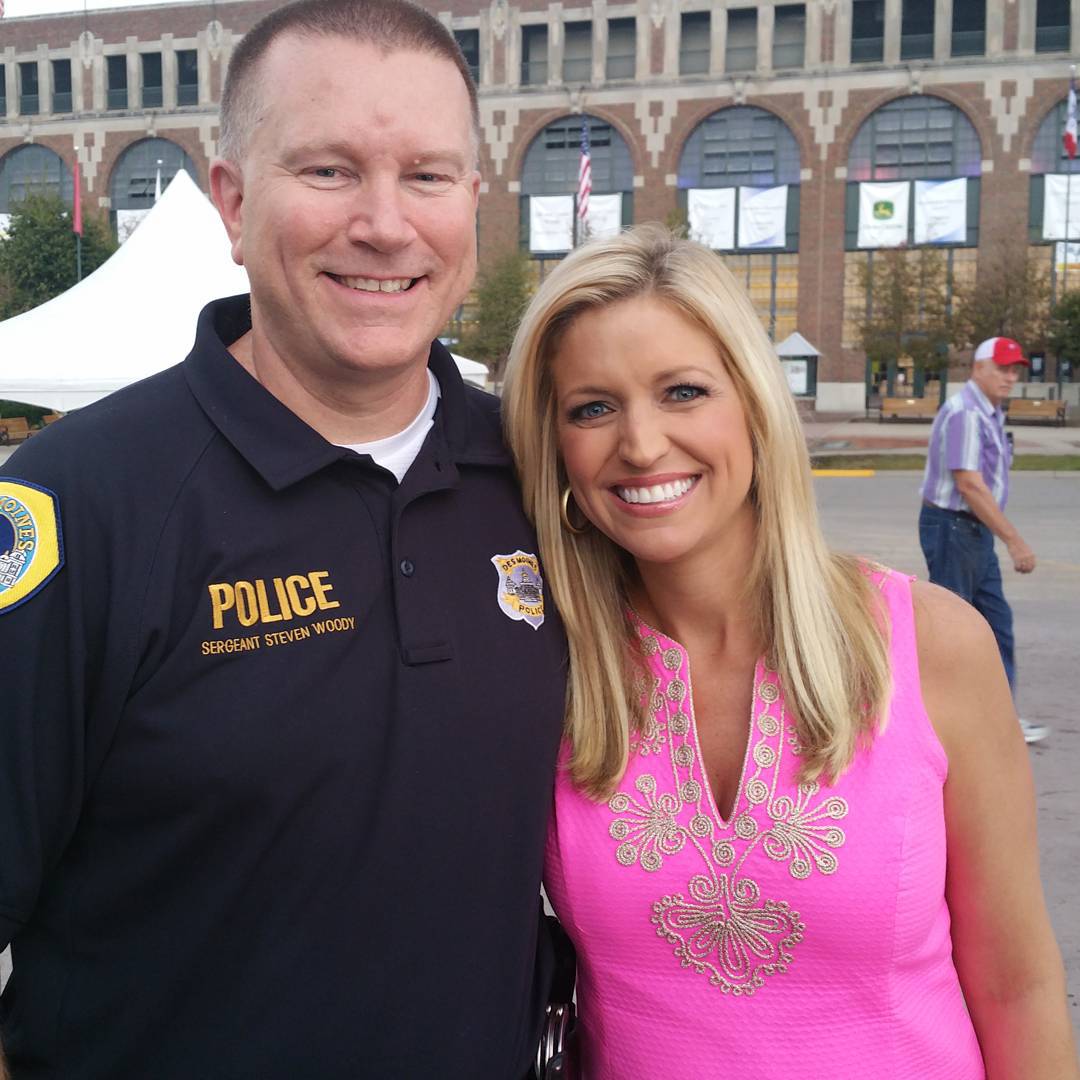In the center of the image, a man and a woman are posing and smiling directly at the camera. The man, with a short buzz cut, is wearing a black police polo shirt with a yellow "Police" text on one side and a badge illustration on the other. The shirt also features the name "Sergeant Stephen Woody." He has his arm around the woman next to him, who has short straight blonde hair and is dressed in a pink tank top with white embroidery. The setting is outdoors, likely in the middle of the day, as there is ample natural light. 

They are standing on an asphalt road with a sidewalk beneath it, and in the background, there's the façade of a brown stadium adorned with a couple of signs. Further details include a white tent visible behind the stadium and an older man in shorts and a red hat photobombing in the distance. He is wearing white sneakers and appears to be looking at the couple from afar. The overall scene is bustling with colors, including shades of pink, tan, brown, blue, black, yellow, and purple.